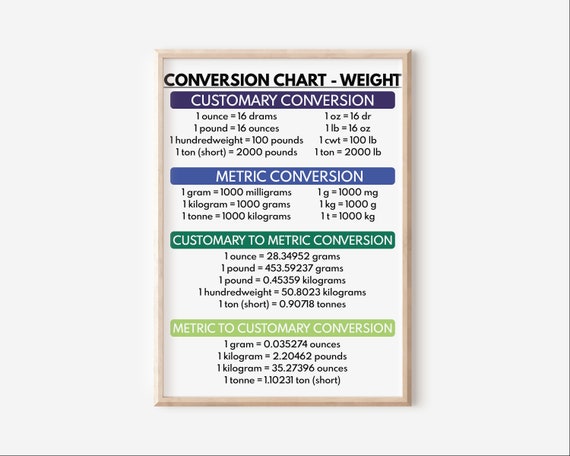This image features a detailed conversion chart prominently displayed in the center, encased in a thin, light brown wooden frame. The chart, set against a plain white background, is divided into several sections for easy reading. 

At the very top, in bold black text, underlined for emphasis, the title reads "Conversion Chart - Weight". Directly below this, within a purple rectangular box with beveled edges and white print, it states "Customary Conversion". This section lists conversions in black text: "1 ounce (oz) equals 16 drams (dr), 1 pound (lb) equals 16 ounces (oz), 1 hundredweight (cwt) equals 100 pounds (lb), and 1 ton (short) equals 2,000 pounds (lb)". The same conversions are reiterated using abbreviations.

Beneath that, a blue rectangle with white print is labeled "Metric Conversion". In this section, the black text lists: "1 gram (g) equals 1,000 milligrams (mg), 1 kilogram (kg) equals 1,000 grams (g), and 1 ton (t) equals 1,000 kilograms (kg)" alongside their abbreviated forms.

Further down, a green rectangle with beveled edges and white print is labeled "Customary to Metric Conversion". It details conversions such as "1 ounce (oz) equals 28.34952 grams (g), 1 pound (lb) equals 453.59237 grams (g), 1 pound (lb) equals 0.45359237 kilograms (kg), 1 hundredweight (cwt) equals 50.80234544 kilograms (kg), and 1 ton (short) equals 907.18474 kilograms (kg)".

At the bottom, within a light green beveled rectangle with white print, it reads "Metric to Customary Conversion". This section includes conversions like "1 gram (g) equals 0.035274 ounces (oz), 1 kilogram (kg) equals 2.20462 pounds (lb), and 1 tonne (t) equals 1.10231 US tons (t)".

The overall background of the image is light gray, framing the detailed and colorful sections of the conversion chart.